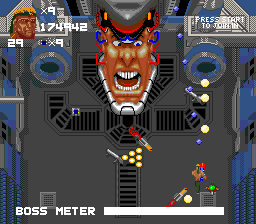The scene features a Boss Meter displayed at the bottom left, titled "Boss Base Meter," with a very large white rectangle beside it. In the top-left corner, an image of a stoic man with a black bandana and yellow hair is shown. The bottom left displays the number "29," while the bottom right indicates "x9," emphasizing the high difficulty level. At the center-bottom, the numbers "174942" are prominently visible.

On the far right, the text "Press Start to Join" invites participation. The ground is primarily gray. On the left side, there is a gray cannon adorned with blue circles and a black center. Both the left and right walls are mostly blue. The bottom right depicts a character shooting, who is wearing a bandana.

At the very top, a large, menacing face is visible with a metal chin, blue and red wires protruding from the face, an open mouth displaying teeth, and an overall angry expression. The figure is wearing a metal cap with a red hood and black rim.